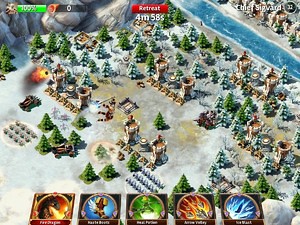The image appears to be a screenshot from an old real-time strategy video game, characterized by an isometric top-down view. The scene captures a snowy landscape with a blue river meandering across the top-right corner, surrounded by pine trees and various military structures, including towers, bases, and catapults launching flaming projectiles. Troops are lined up in equally spaced rows, ready for battle.

Notable interface elements are present on the screen: At the top-left corner, a green health bar displaying "100%" is visible, while the top center reads "Retreat" followed by a countdown timer set to 4 minutes and 58 seconds. In the top-right corner, the name "Chief Sigvard" is displayed. Additionally, symbols and buttons related to game abilities or attacks are arrayed along the bottom of the screen. These include, from left to right, a red icon depicting a fire-breathing dragon, a blue icon with a winged boot (likely Icarus' winged shoes), a green circle, a red icon with arrowheads flying in, and a blue icon showing an ice burst with shards of ice scattering. These icons represent different abilities or actions players can perform within the game.